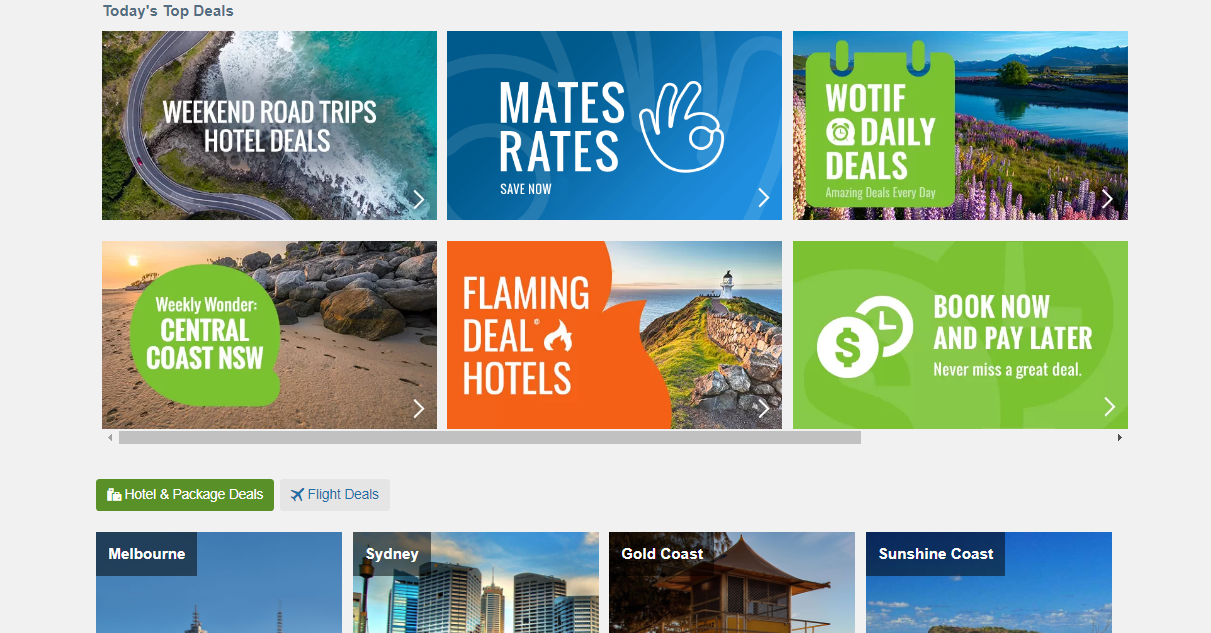The webpage features a gray background adorned with various rectangles, each containing distinct, visually appealing content. At the top left, dark gray text announces "Today's Top Deal." Below, an image depicts a winding road through light and dark green hills adjacent to a cyan-blue waterway with snow-capped waves. Overlaying this picturesque scene, bold white text reads "Weekend Road Trips."

Next, there's an image of a tan and brown beach, strewn with rocks in varying shades ranging from gray and bluish-gray to brown. Footprints are visible in the sand. Over this, a slightly oblong green circle bears the white text "Weekend Wonder," followed by bold white text stating "Central Coastal NSW."

On the right side, a blue square with bands of gray or light blue sits, featuring bold white text that reads "Mats Rates" and "Save Now," accompanied by an 'okay' hand symbol.

Further right, there is an image of a serene waterway bordered by trees, with the blue water reflecting a clear blue sky. A mountain range and colorful flowers (purple, pink, and red) adorn the background. Over this, a green calendar icon with white text reading "WOTIF" is displayed, followed by a clock icon and bold white text announcing "Daily Deals." Below, smaller white text promises "Amazing deals every day."

Another image showcases a white lighthouse perched on a ridge near a vast, blue water body, possibly a lake or ocean, with an orange-tinted sky suggesting a sunset. Surrounding the lighthouse are brown and tan rocks, with green grass on either side. Bold white text across the image reads "Flaming Deal Hotels," with a flame icon next to "Deal," set against an orange background.

The final section features a white circle with a green money symbol and a clock icon; the clock's hands and outline are white, set on a green background. Bold white text encourages "Book Now and Pay Later," while smaller, non-bold text advises "Never miss a great deal," accompanied by a bold white arrow to the right.

At the very bottom, a navigation bar contains a sliding dark gray rectangle, flanked by black arrows on the left and right for easy maneuvering.